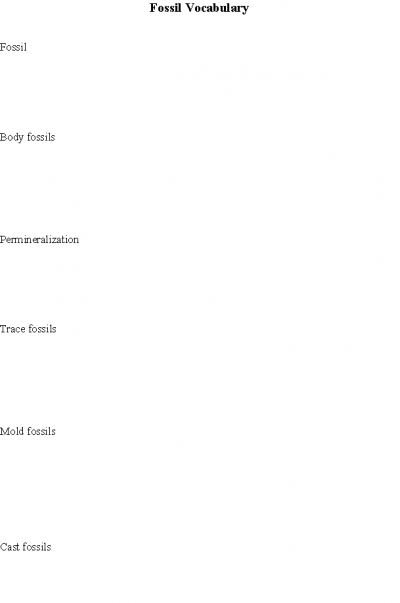The image depicts a straightforward and minimalist page centered around fossil vocabulary. The page predominantly features a header at the top, showcasing the title "Fossil Vocabulary" in bold, black font on a white background. Each segment beneath the header lists different types of fossils, separated by approximately an inch and a half of white space.

The listed terms, starting from the top and moving down in a single column on the left-hand side, are as follows:
1. **Fossil**
2. **Body Fossils**
3. **Permineralization**
4. **Trace Fossils**
5. **Mold Fossils**
6. **Cast Fossils**

These terms are printed in a smaller, finer gray font that contrasts with the bold header, signifying their auxiliary role in the context of the page. The arrangement suggests that additional information may be written in the future, making it a clearly structured and educational outline on fossil terminology.